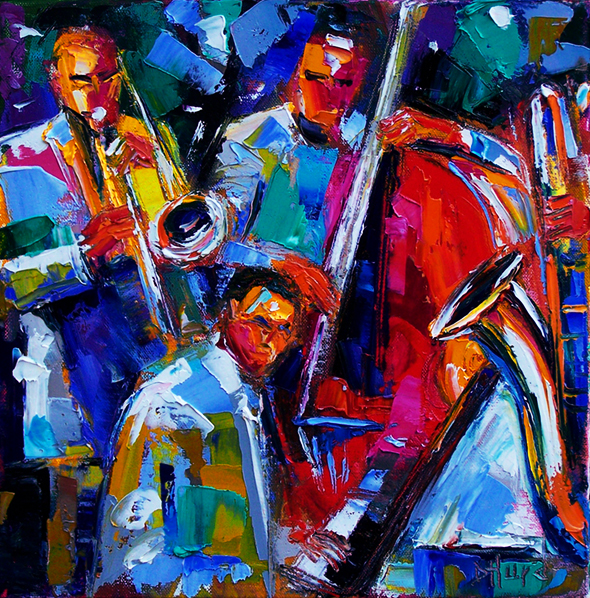The image is a square, colorful, and abstract painting, possibly reflecting an abstract impressionist style. The scene depicted appears to be a lively jazz band immersed in their performance, rendered in vibrant and vivid hues, including blues, reds, yellows, greens, and pinks. The composition features three prominent musicians: on the top left, a man playing a trombone; next to him, another individual handling a large wooden bass; and in the foreground, a seated pianist deeply engaged with his instrument, his head raised as if reading music. Additionally, on the far right, only the saxophone and the hand of another player are visible. The painting showcases bold and blocky forms with an energetic interplay of colors, capturing the dynamic atmosphere and movement of the jazz session. The signature "DH" along with other indistinguishable letters is carved into the paint at the lower right corner of the piece.